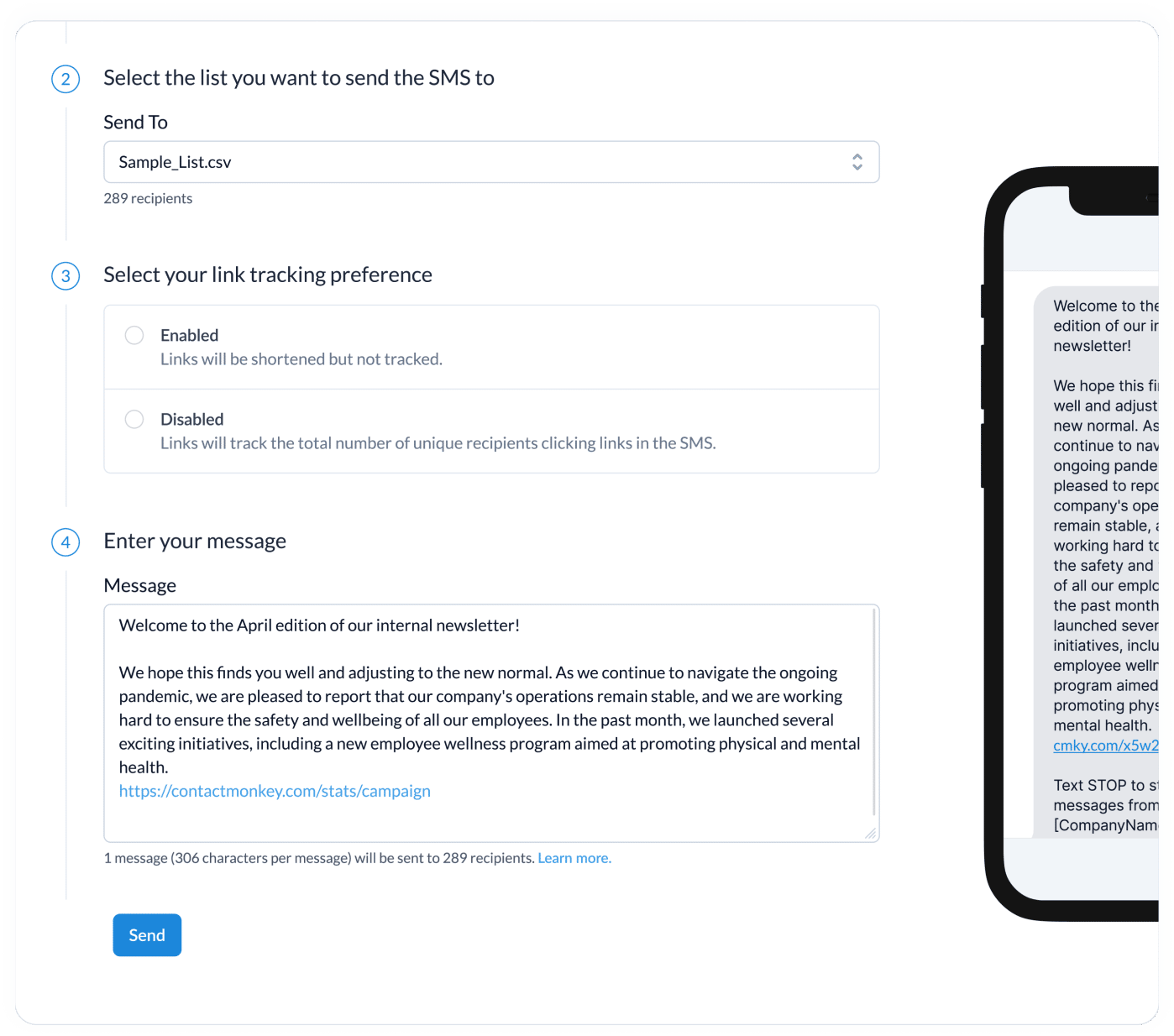A detailed screenshot of a messaging interface intended for sending SMS notifications is on display. On the left side, occupying the majority of the image, is the main input area with several step-by-step options. At the top, a heading reads "Select the list you want to send an SMS to," followed by a drop-down menu currently displaying "sample," indicating a list of 289 residents.

Below this, sequentially numbered options (2, 3, and 4) are listed vertically. The second option asks the user to "select your link tracking preference," with toggles to enable or disable tracking. The third step prompts the user to "enter the message," presenting a sample paragraph related to an April newsletter, discussing the "new normal" during a pandemic. This sample message includes a URL link at the bottom.

The screen's fourth section informs the user that "one message will be sent to the recipient." At the very bottom of this interface, a blue "Send" button is prominently placed.

To the right of the interface is a cropped screenshot of a smartphone display. The partial view shows a message pertaining to welcoming recipients to a newsletter SMS, though much of the text is cut off, rendering some of the content unreadable. The phone image overlaps slightly with the main interface, suggesting this segment is related contextually to the input fields on the left. This setup appears specifically designed for sending mass SMS updates to a predefined list.